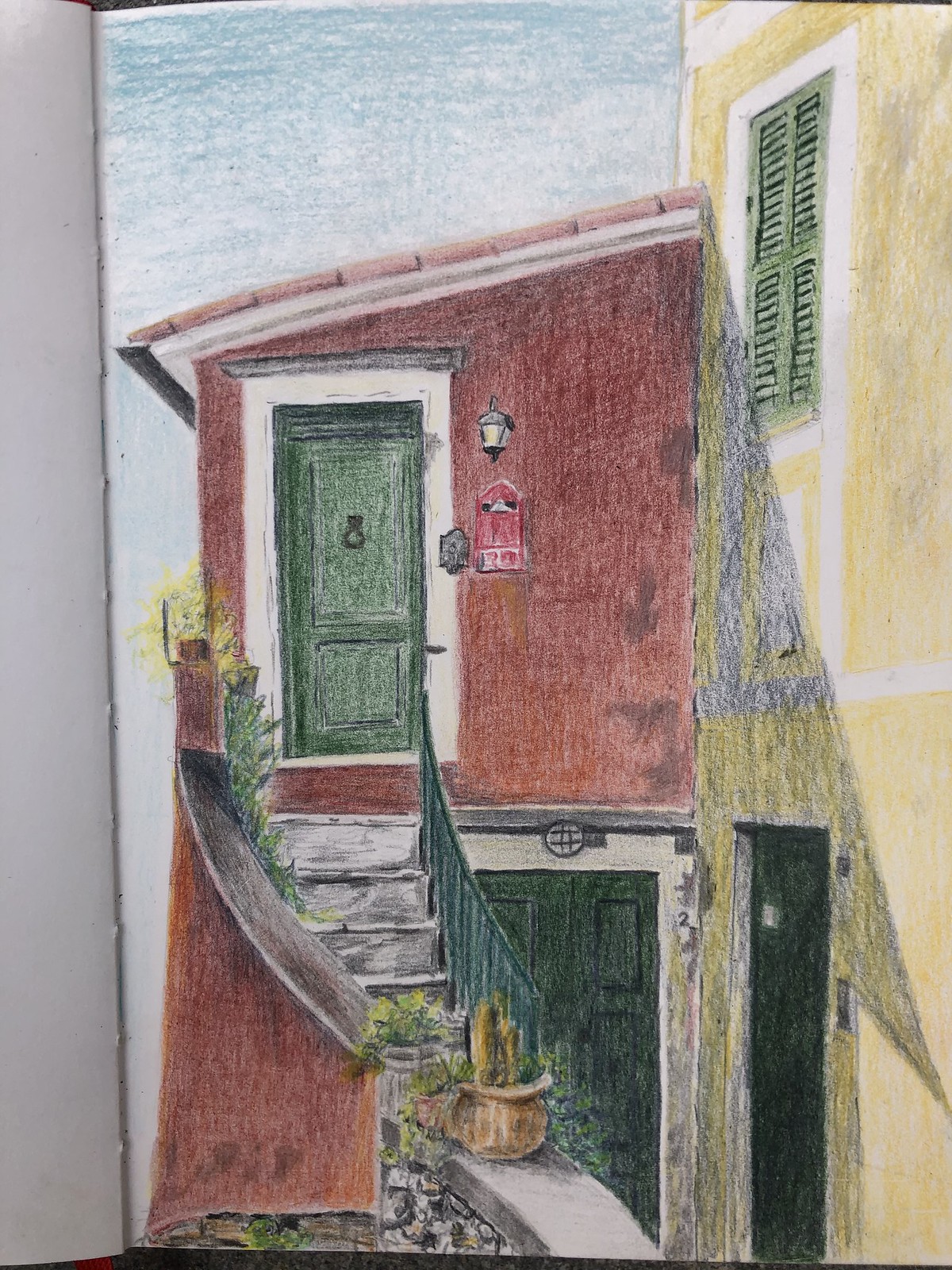This vibrant drawing illustrates a charming home adorned in various colors. The primary house is rendered in a deep red hue, prominently displaying the number "120" near a small mailbox, which seems perfect for dropping letters or even tiny pieces of melon. The home's green door is framed by a crisp white exterior, with a light fixture illuminating the entrance.

A small staircase descends to reveal what appears to be a second unit, also furnished with a green door. Adjacent to the red house stands a yellow building, characterized by its white and green windows. The sky above is a bright blue, suggesting a sunny day.

Flourishing plants add a touch of nature to the scene, enhancing the overall appeal of the drawing. The artistic style hints at the use of crayons or colored pencils, showcasing impressive detail and vibrancy. Overall, it's a wonderfully executed piece, rich in both color and charm.